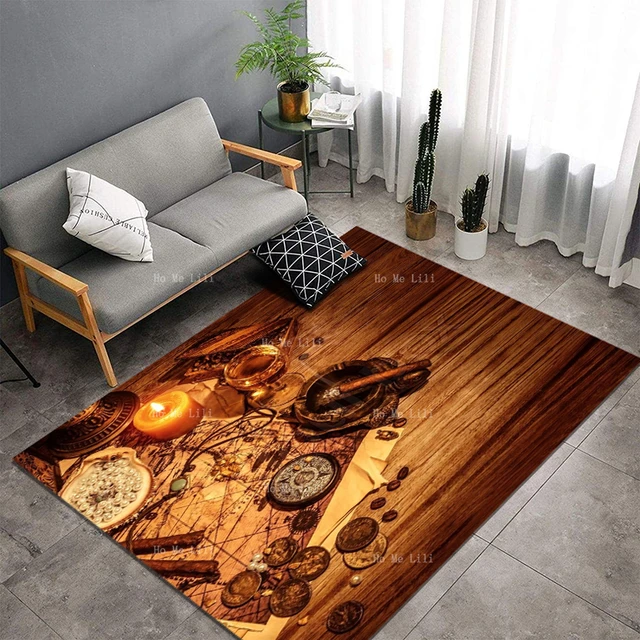An aerial view captures a cozy living room scene featuring a gray couch with a white striped pillow. Below, a black and white striped pillow rests on a rug that mimics a wooden design, adorned with images of everyday objects such as watches, candles, and a cigar. A round circular table with a large plant stands nearby, while various other plants and cactuses in gray and white pots add greenery to the space. Long white curtains cover the windows on the right side, and additional decor includes wooden and copper bowls. The floor itself is wooden, with gray tiles also present, providing a harmonious mix of textures and colors in this inviting environment.